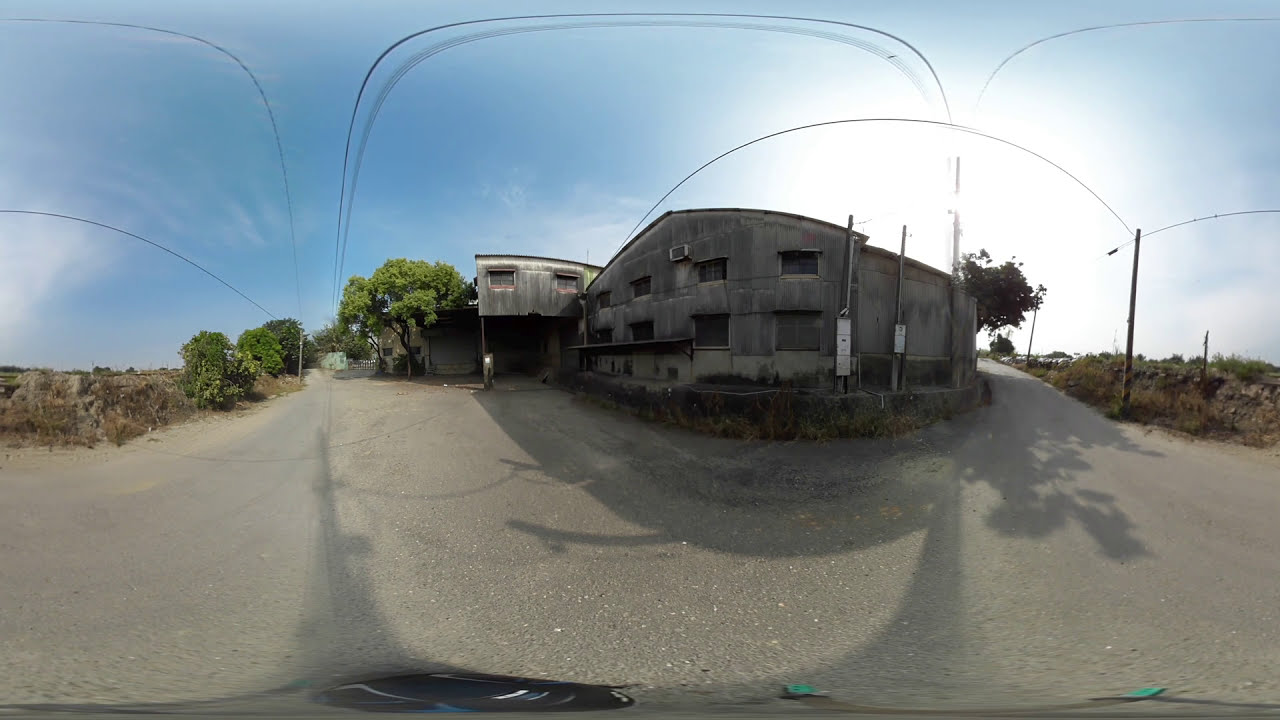This image depicts a distressed and vacant gray building that appears to be made out of heavy concrete or cement. The dingy structure, possibly an old barn or abandoned industrial facility, has a worn exterior with weather-beaten siding that might have once been beige but now looks more gray. The main building, standing a couple of stories high, features boarded-up windows and an attached carport. There’s also a partially elevated section that suggests a secondary floor or back office area beneath which a car could potentially be parked.

In the foreground, an extensive area of macadam or asphalt stretches out, creating what looks like a driveway or parking area devoid of any vehicles. The road or path leading up to the building appears gray and paved, although the distorted nature of the image makes it difficult to distinguish its material clearly.

On the left, sparse and dying grass is interspersed with patches of dirt and a scattering of trees. A telephone pole to the right of the building has wires stretching out in arch shapes across the sky, adding to the desolate and neglected atmosphere.